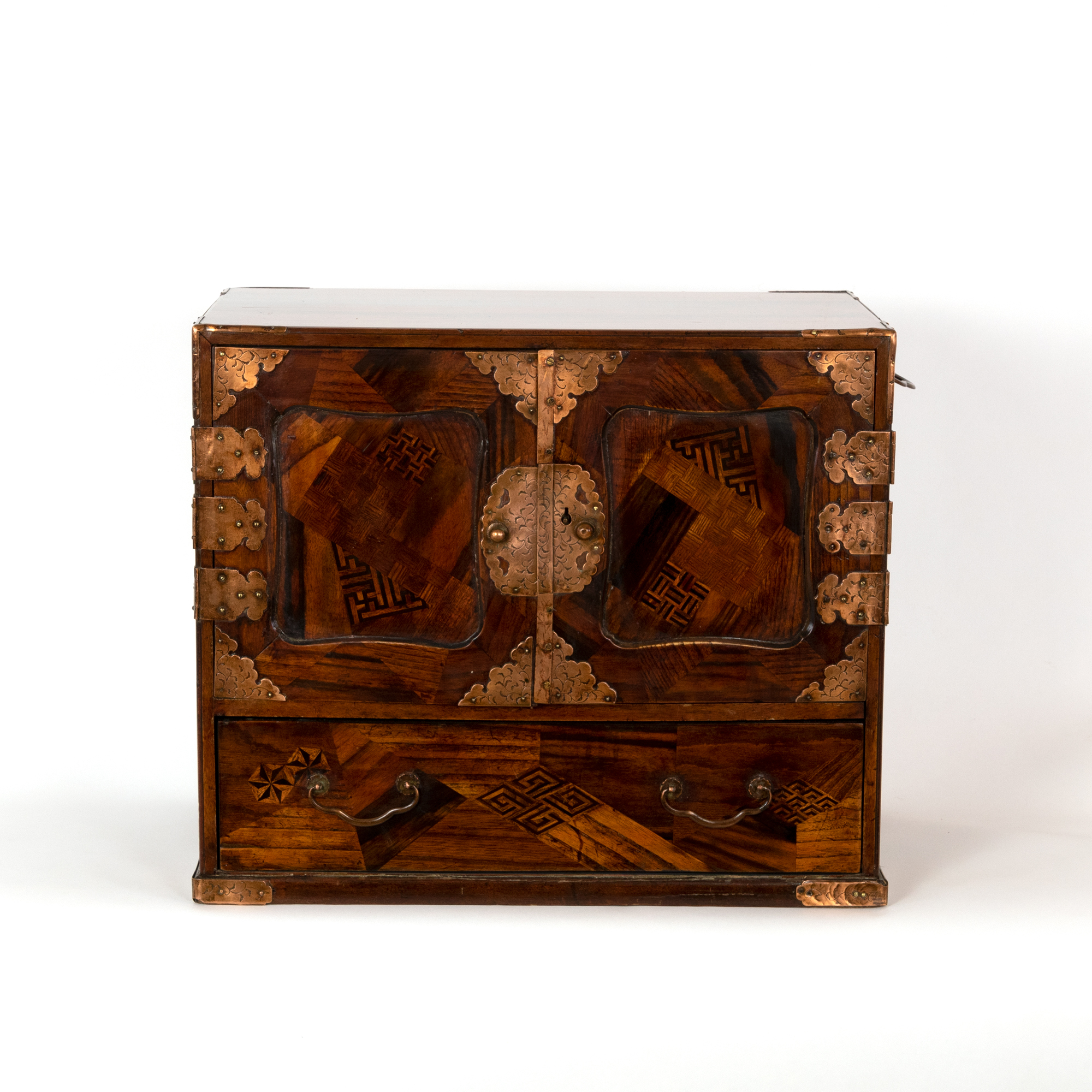This image features a vertical rectangular antique jewelry box set against a very light gray, almost white background. The box itself is crafted from various shades of dark brown wood, giving it a rich, textured appearance. The piece is divided into two main sections. The lower section houses a pull-out drawer, approximately six inches in height. This drawer is fitted with two arch-shaped handles made of dark brown metal.

Above the drawer sit two cabinet doors that open outward. These doors are adorned with intricate decorations: each outer corner features a triangular, jagged-edge dark gold plate, and three rectangular-to-triangular shaped dark gold hinges run down each side. The center of the doors holds small circular knobs, mounted on vertical oval-shaped dark gold plates.

The craftsmanship of the jewelry box is further highlighted by its detailed woodwork, including star and diamond patterns inlaid into the wood. Copper or bronze-colored hinges and guards add a touch of antiquity and elegance, enhancing the overall intricate design of this ornate piece.